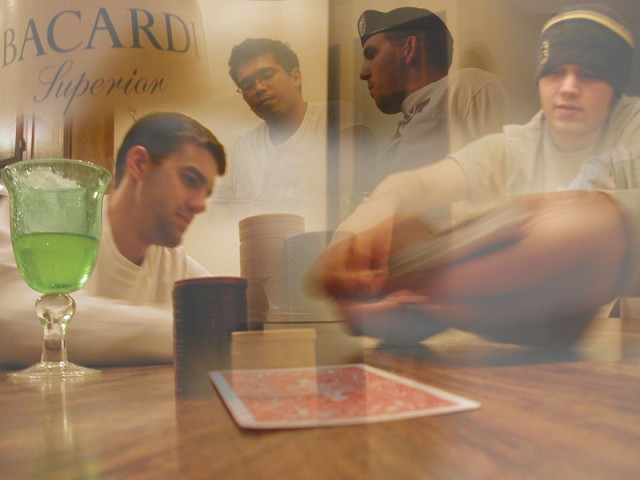A meticulously crafted advertisement for Bacardi Superior sets a somber and introspective scene, deviating from typical party-driven narratives often associated with the brand. In the foreground, a rustic wooden table serves as the centerpiece, adorned with an array of objects that paint a vivid story. A single card from a standard deck, marked by a striking red graphic, lies flat, accompanied by four unevenly stacked piles of poker chips. A distinct goblet cup with a clear base and elegantly green glass-blown body, partially filled with an unidentified liquid, adds a touch of sophistication to the tableau.

The atmosphere is further enriched by an ethereal visual effect reminiscent of TV specters, where the figures of four men are rendered hazy, almost ghostly, yet still discernible. The spectral effect lends an otherworldly tone to the image, drawing the viewer into a contemplative mood. Each of the men, captured in their own activities, contributes to the diverse tableau: one appears in a military uniform, another in the midst of dealing cards, a bespectacled man emanating a solemn air, and a fourth, possibly of Asian, Middle Eastern, or Indian descent, seated in a long-sleeved shirt, mirroring the solemnity of his companions.

Despite being an advertisement for Bacardi, prominently highlighted at the top with the label "Bacardi Superior," the expressions and body language of the men depart from the brand's usual jovial imagery. The ad masterfully juxtaposes the lively expectation tied to Bacardi with a powerful, introspective ambience, capturing a moment heavy with thought and reflection rather than celebration.